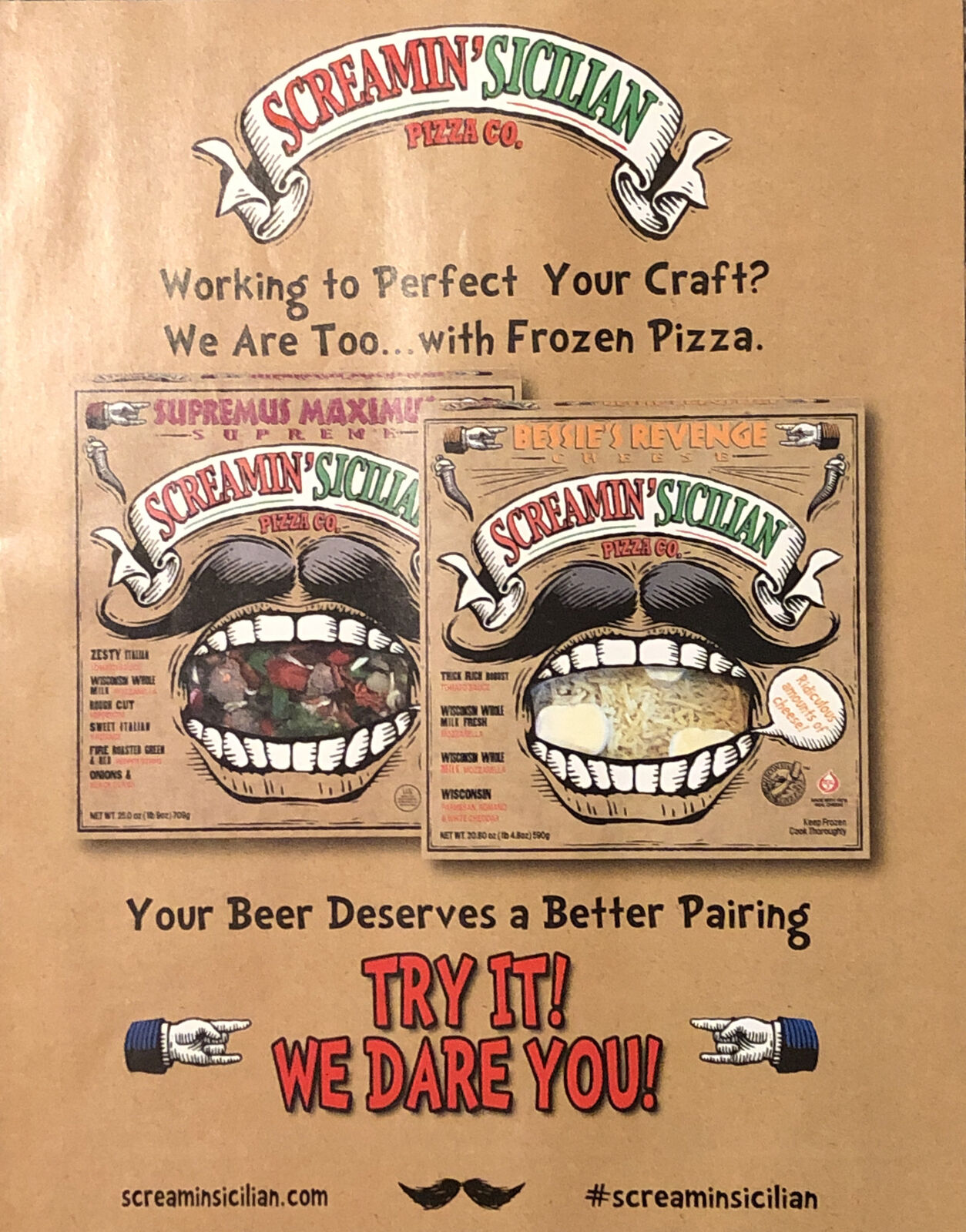This full-page glossy advertisement for the Screamin' Sicilian Pizza Company features a vibrant and engaging design aimed at showcasing their frozen pizza offerings. The ad is dominated by a visually striking poster-like object with the brand name "Screamin' Sicilian Pizzico" prominently displayed at the top on a ribbon arch. Central to the design are stylized cartoonish pizza box images, each featuring a human mouth with a dark black mustache, seemingly screaming, a playful homage to the brand's name.

The advertisement invites pizza lovers with the bold slogan, "Working to perfect your craft? We are too, with frozen pizza," and emphasizes an irresistible challenge with, "Your beer deserves a better pairing. Try it, we dare you," highlighted by two pointing hands. 

Two distinct pizza varieties are showcased: "Supremus Maximus," loaded with an array of toppings akin to a supreme pizza, and "Bessie's Revenge," which promises an indulgence of cheese. Additional callouts include the website, ScreaminSicilian.com, and the hashtag #ScreaminSicilian beneath a mustache illustration, drawing focus to their online presence. This detailed ad not only visually entices but also cleverly associates the brand with both quality and personality, encouraging consumers to give their pizzas a try.